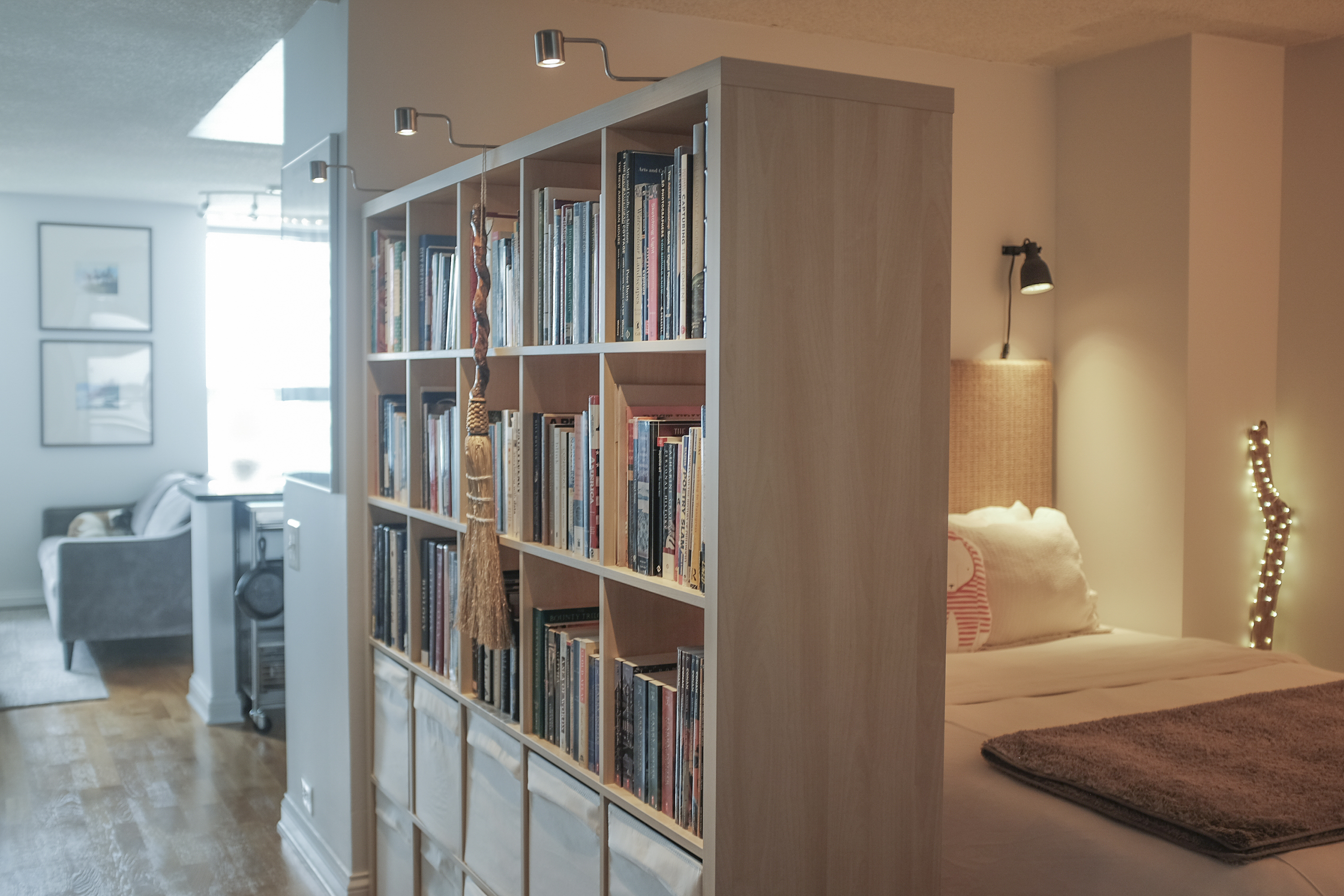This photograph captures the interior of a bright, modern loft apartment with an open-concept design. The main feature is a large, wooden bookshelf that functions as a room divider, separating the living area from the bedroom. The bookshelf, filled with various books and adorned with small lamps, acts as a makeshift wall, providing privacy for the bedroom, which is situated behind it. The bedroom area has beige walls, is softly illuminated, and includes a bed with white pillows and sheets.

On the left side of the bookshelf, the open living space includes a cozy area with a couch, a small rug, and gray chairs. The windows in the living room allow plenty of natural light to flood the space, enhancing its bright and welcoming ambiance. The walls in this section have white paintings or pictures adding to the decor. Adjacent to the living space is a kitchenette, marked by a slight counter that further defines the room's functionality.

The apartment floor is primarily wooden, contributing to its modern aesthetic. Overall, the image showcases a seamless blend of living, cooking, and sleeping areas within a thoughtfully designed small-space layout.